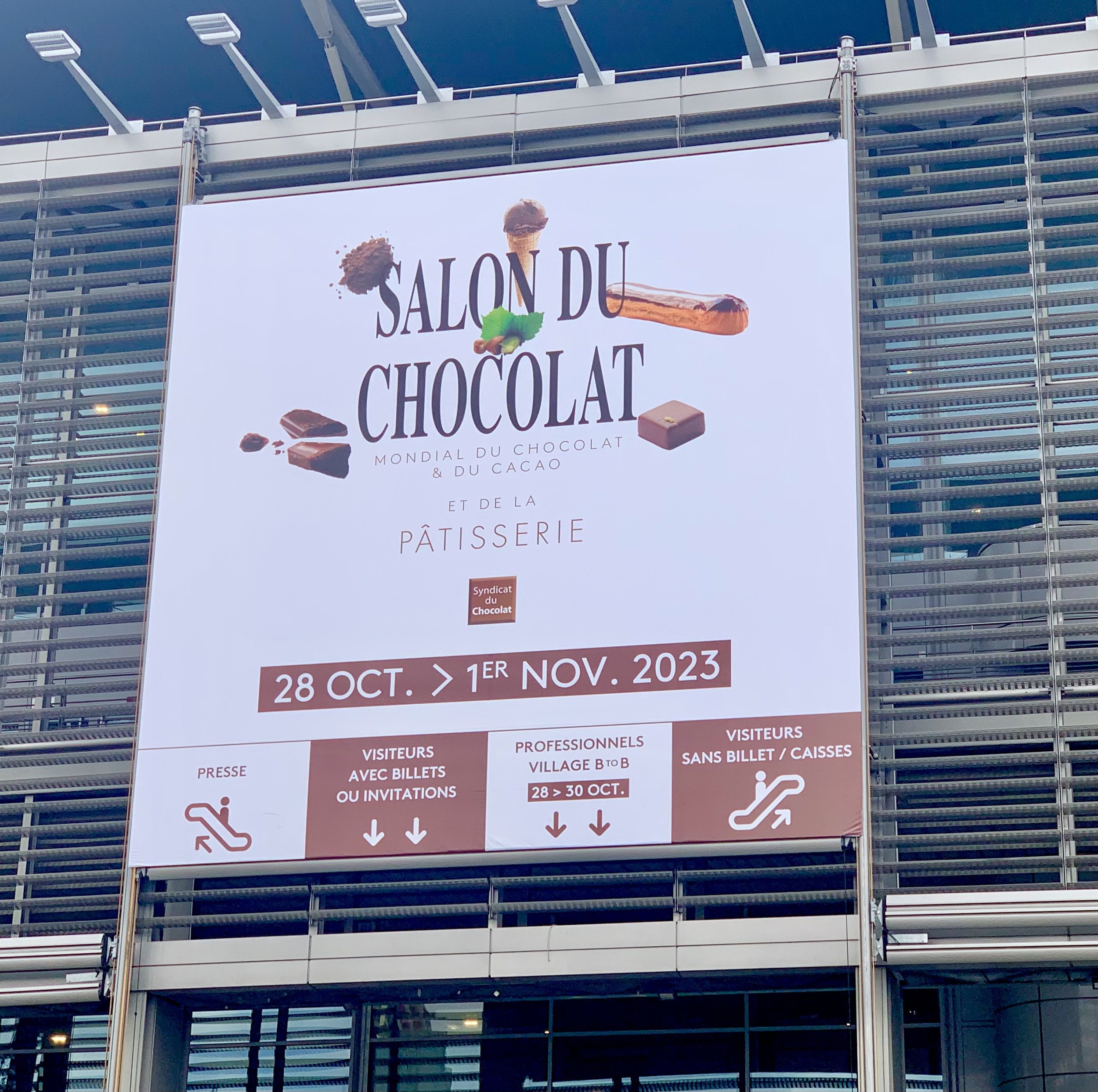The image depicts a large banner hanging in front of a building with metal paneling and slatted shades. The banner prominently displays "Salon du Chocolat" in large, blue, capital letters. Surrounding this title are various images featuring chocolate treats such as eclairs, brownies, and a chocolate ice cream cone. Beneath the title, French text mentions "patisserie" and other details, indicating it's for a chocolate festival. The banner specifies the event dates as October 28th to November 1st, 2023. Below this, the poster details four different entry lines for the press, visitors with invitations, visitors without invitations, and professionals, depicted through a mix of text and icons. In addition, directional arrows and elevator icons suggest access information, all formatted within alternating white and brown squares.